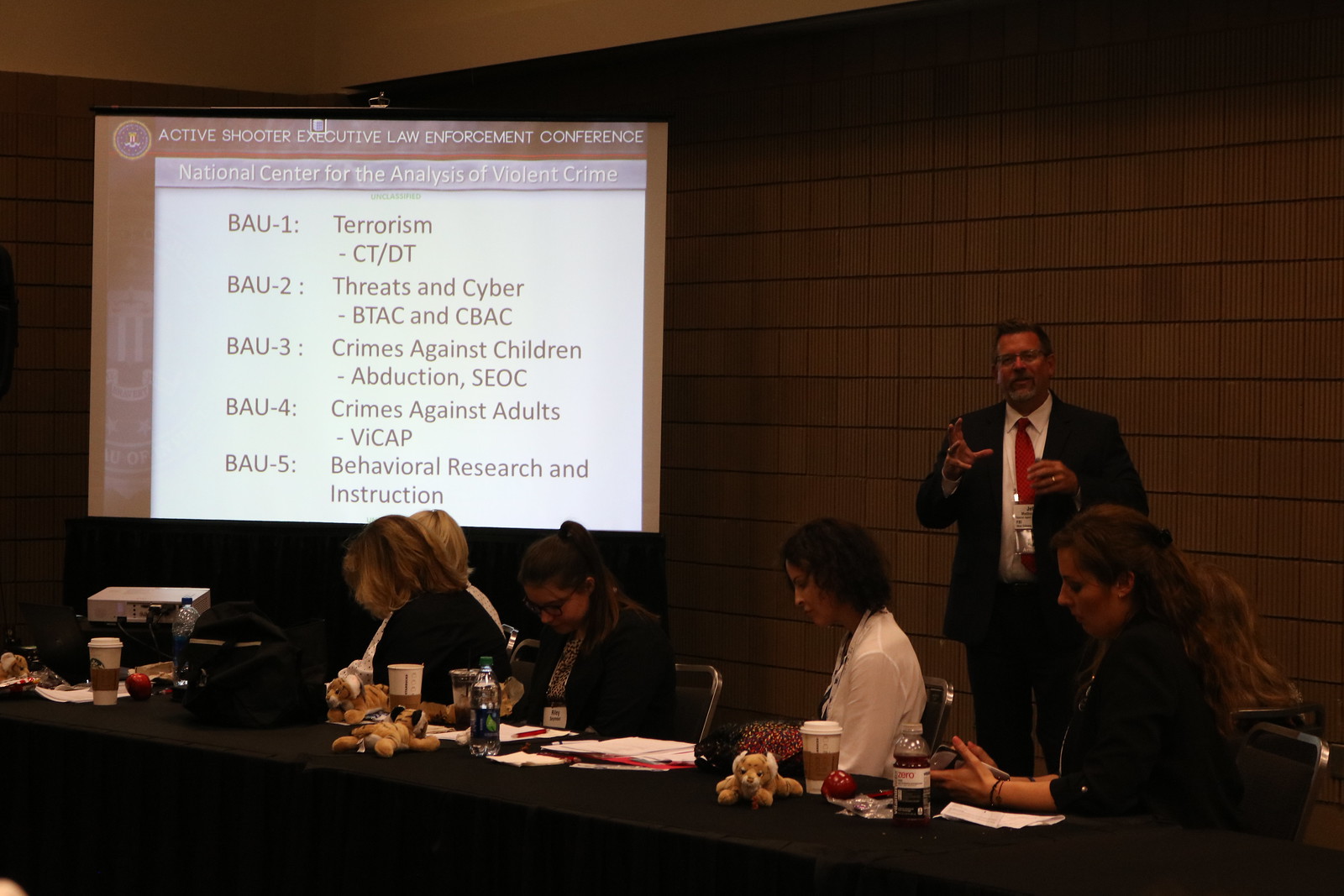The image depicts a man delivering a presentation at the "Active Shooter Executive Law Enforcement Conference," organized by the National Center for the Analysis of Violent Crime. The man, dressed in a black suit with a white shirt and red tie, stands against a textured stone wall on the right side of the image. He is gesturing with his right hand toward a projector screen to his left, which displays the conference title and an emblem. The screen also lists various topics covered at the conference, including terrorism, threats and cyber issues, crimes against children, crimes against adults, and behavioral research and instruction, designated by specific BAU and BTAC/CBAC codes. In the foreground, four to five women are seated at a black-draped table, engrossed in documents, laptops, or smartphones, with fruit and drinks also visible. The overall setting appears to be a formal meeting space such as a City Council or school board meeting.